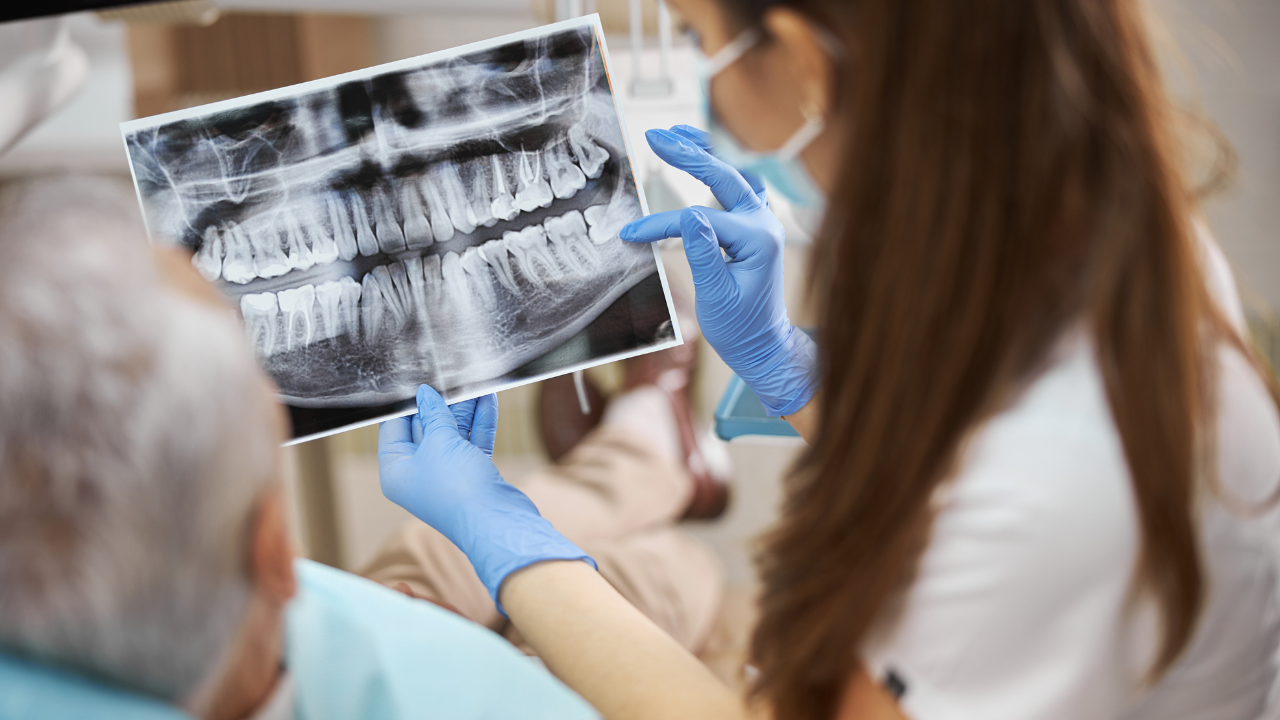In this detailed color photograph, a female dental professional, possibly a dentist or dental assistant, with reddish-brown, slightly messy hair, is captured mid-consultation. She is wearing a white medical coat, a blue face mask, and blue latex gloves. She's holding a black-and-white panoramic dental x-ray, showing a full set of teeth, including the impacted wisdom teeth of an older male patient with gray hair. The man's head is visible as he reclines in the dental chair, donning a dental bib. His white hair contrasts with the tan and white hues of the blurred background, which features some indistinct office furniture. The professional is pointing at a specific area on the x-ray, with her right index finger extended, directing the patient's attention to the condition of his teeth. The image primarily highlights the interaction over the dental x-ray amidst a clinical setting, with dominant colors being light blues, red-brown for the hair, white, and the grayscale of the x-ray.